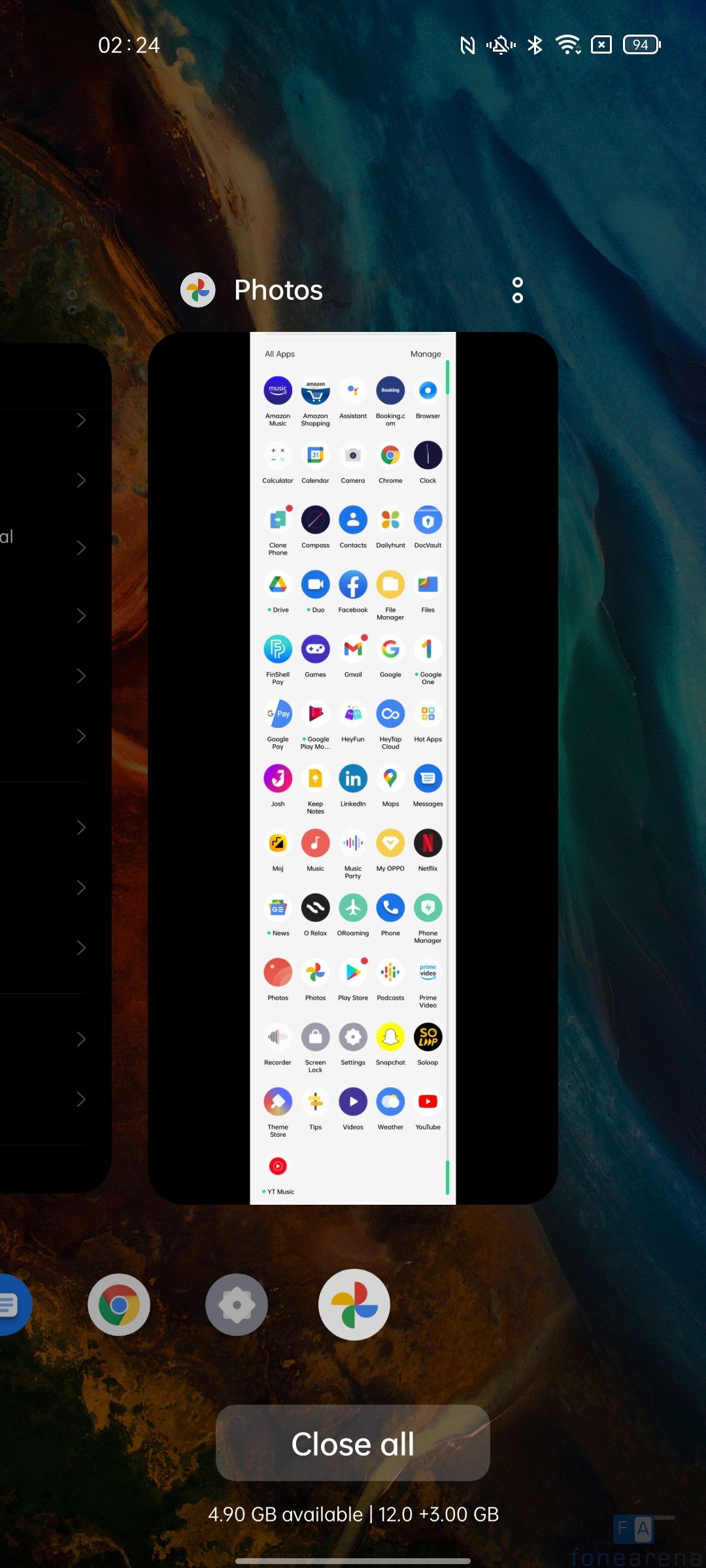The image showcases the home screen of an Android device, either a tablet or a phone. In the upper left corner, the time is displayed as "02:24" in white text. Moving rightward, a sequence of status icons typical of Android devices is visible: 

1. An outlined "N" indicating a notification.
2. A bell with a slash through it, signifying silenced notifications.
3. The Bluetooth symbol.
4. The WiFi symbol.
5. An outline of a SIM card with an "X" marking no SIM card present.
6. A battery icon displaying "94%" to indicate the battery level.

Beneath this status bar is a rectangular window with the "Photos" label, accompanied by the Google Photos logo towards the right. Two outlined white dots lie adjacent, and the background is black transitioning to an off-white or gray area populated with numerous circular app icons. Among these icons, the Google, Gmail, Discord, Facebook, and Drive apps are notably present, suggesting common applications used by the user.

At the bottom center of the device's screen, the Google Photos logo reappears. Leftward is a gear icon indicating the settings menu, followed by the Google Chrome icon, and further left, a blue icon with a message bubble representing the messaging app. At the very bottom, a rounded rectangular button labeled "Close All" in white is centrally placed.